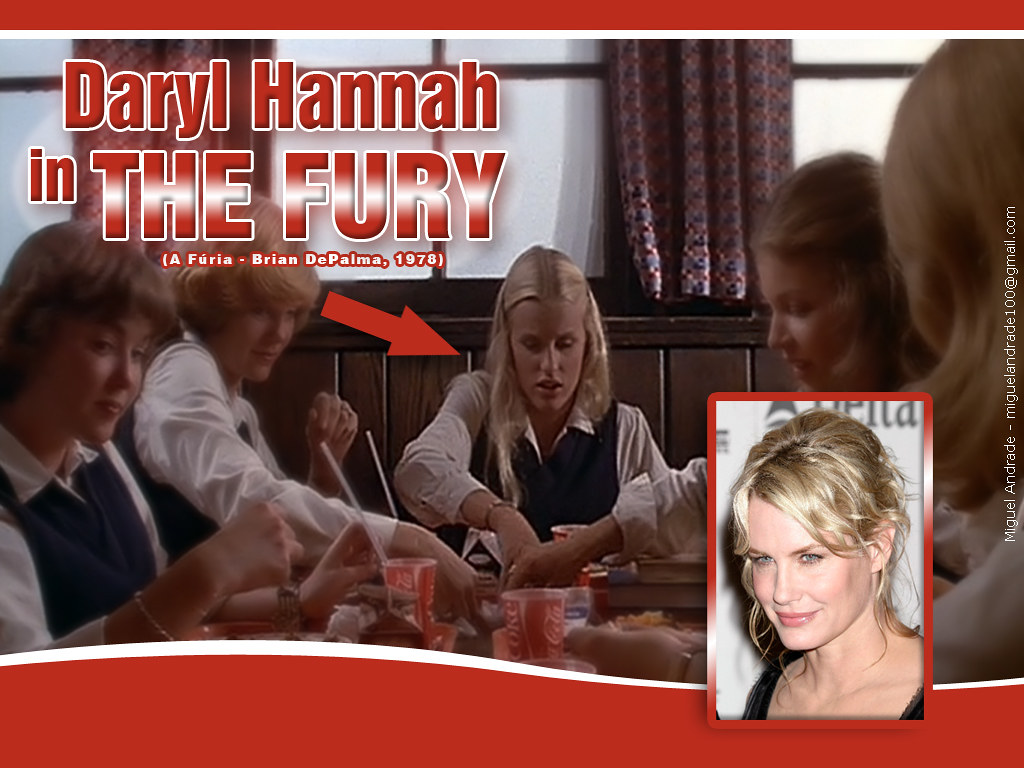The image depicts a scene from what appears to be a film, likely "The Fury" directed by Brian De Palma in 1978. Centered in the picture are several women seated at a table in a restaurant setting, identifiable by Coca-Cola cups and food items on the table. The women, dressed in coordinated schoolgirl outfits featuring white collared shirts and black vests, have 1970s hairstyles. A red arrow prominently highlights one blonde woman among them, identified by the accompanying text, "Daryl Hannah in The Fury," with further details reading "A. Fuhrer, Brian De Palma, 1978." In the upper left of the image, the text is framed with a red and white outline. Additionally, in the bottom right corner, there's a contemporary photo of a blonde woman, presumably Daryl Hannah, with blue eyes and an older appearance. Along the image's right vertical edge, there's a watermark in white text, "Miguel Andrade 100 at google.com."